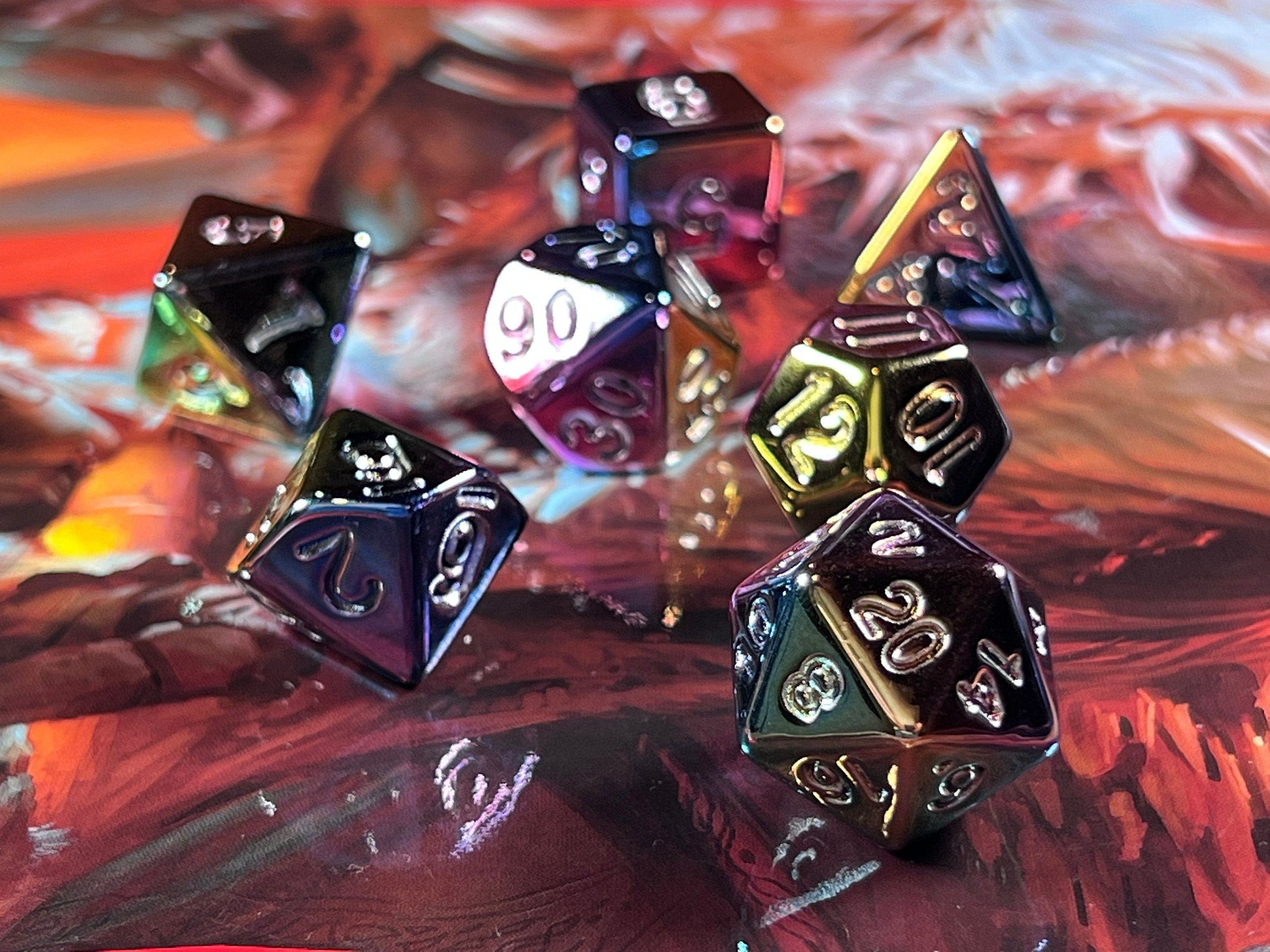This image showcases a vibrant collection of iridescent, multi-sided dice scattered on a patterned tabletop with hues of red, orange, and purple. The closest die, which is silvery in color, reveals the numbers 2, 20, 14, 8, 16, and 6. To its left, a die displays the number 6 and 2 upside down, with the 9 right side up. Nearby, another die shows the numbers 90 and 30, although the rest are obscured. Further back, a die presents the numbers 12, 10, and 11, positioned beside a distinctive triangular die and a square die, with their numbers hidden. Off to the left, another die prominently features the number 5. These dice, reflecting various shades of purple, yellow, green, and blue, capture and illuminate the surrounding light, adding to their enchanting appearance. The background is muted and blurry, emphasizing the colorful, shiny dice and enhancing the overall aesthetic of this captivating scene.